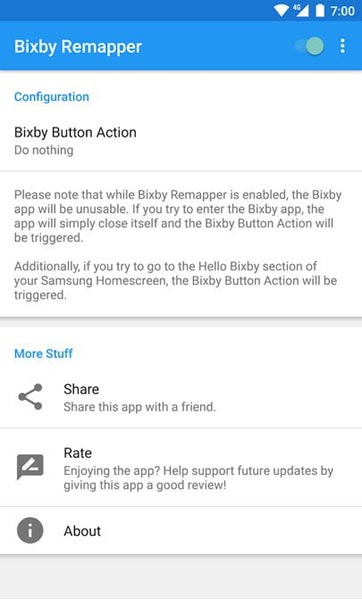The image depicts a smartphone screen with a predominantly blue interface at the top and a white background beneath it. At the very top, a dark to medium blue strip displays icons indicating full Wi-Fi, 4G cellular signal, full battery, and the number "700".

Below this strip, a lighter blue section contains the text "Bixby Remapper" aligned to the left. On the right side of this section, there's a toggle switch currently set to "Off," accompanied by three vertically aligned dots indicating a menu.

The main body of the screen has a white background. To the left, the text "Configuration" is displayed in blue. Below this, the text "Bixby Button Action" is aligned to the left, followed by "Do Nothing" on the next line. A note follows, explaining that while the Bixby Remapper is enabled, the Bixby app will be unusable. It mentions that attempting to enter the Bixby app will close it, triggering the Bixby button action. Additionally, holding the Bixby button in the Samsung home screen will trigger the same action.

A thick gray line separates this section from the next. Below the line, "More Stuff" is written in blue, followed by "Share" and "Share this app with a friend". A thin gray line then separates this from the final text section.

The last portion encourages users to "Rate and Enjoy the App" and help support future updates by leaving a positive review. Below it, there's a section labeled "About" with an icon next to each line of text. The "Share" section is marked with an icon resembling a circle with two lines extending out and ending in circles. The "Rate" section features an icon that looks like a text bubble or comment box.